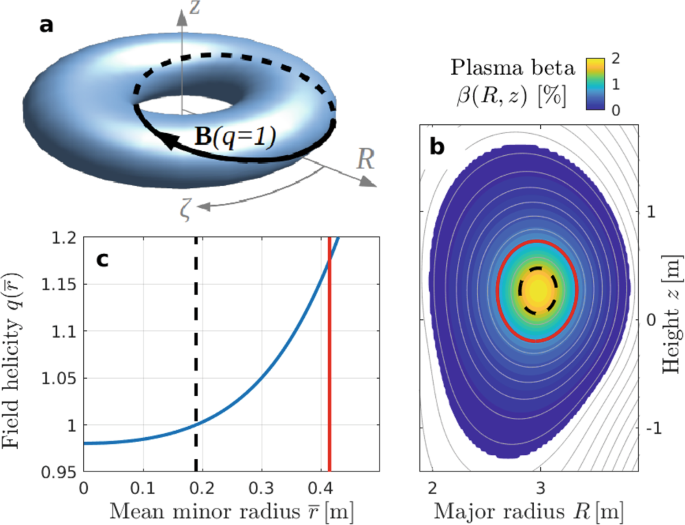The image displays a detailed scientific diagram consisting of three main visual elements. In the top left section is a torus-shaped (donut-shaped) object labeled "A," which is a light blue color. This section includes an advanced mathematical formula: "B(Q=1)" and features several directional arrows. A gray arrow extends vertically through the center labeled "Z," and another horizontal arrow on the right labeled "R" with a smaller arrow featuring a peculiar symbol resembling a "Z" with a squiggly tail.

The section immediately to the right, labeled "B," presents a detailed chart for plasma beta. This chart has a color gradient key, with varying hues indicating different plasma beta values. The X-axis denotes the major radius (in meters), and the Y-axis indicates height (also in meters). The chart is color-coded from dark blue on the outskirts to a yellow center, transitioning through aqua, green, and surrounded by a red line.

The third section, labeled "C," positioned at the bottom left of the image, includes another chart with X and Y axes. The Y-axis is labeled "Field Helicity, Q," while the X-axis specifies the mean minor radius, measured in meters. The plot features a black dotted line at around the 0.2 mark on the minor radius scale, with a blue ascending line from beneath the 1 mark, indicating a relationship between field helicity and mean minor radius.